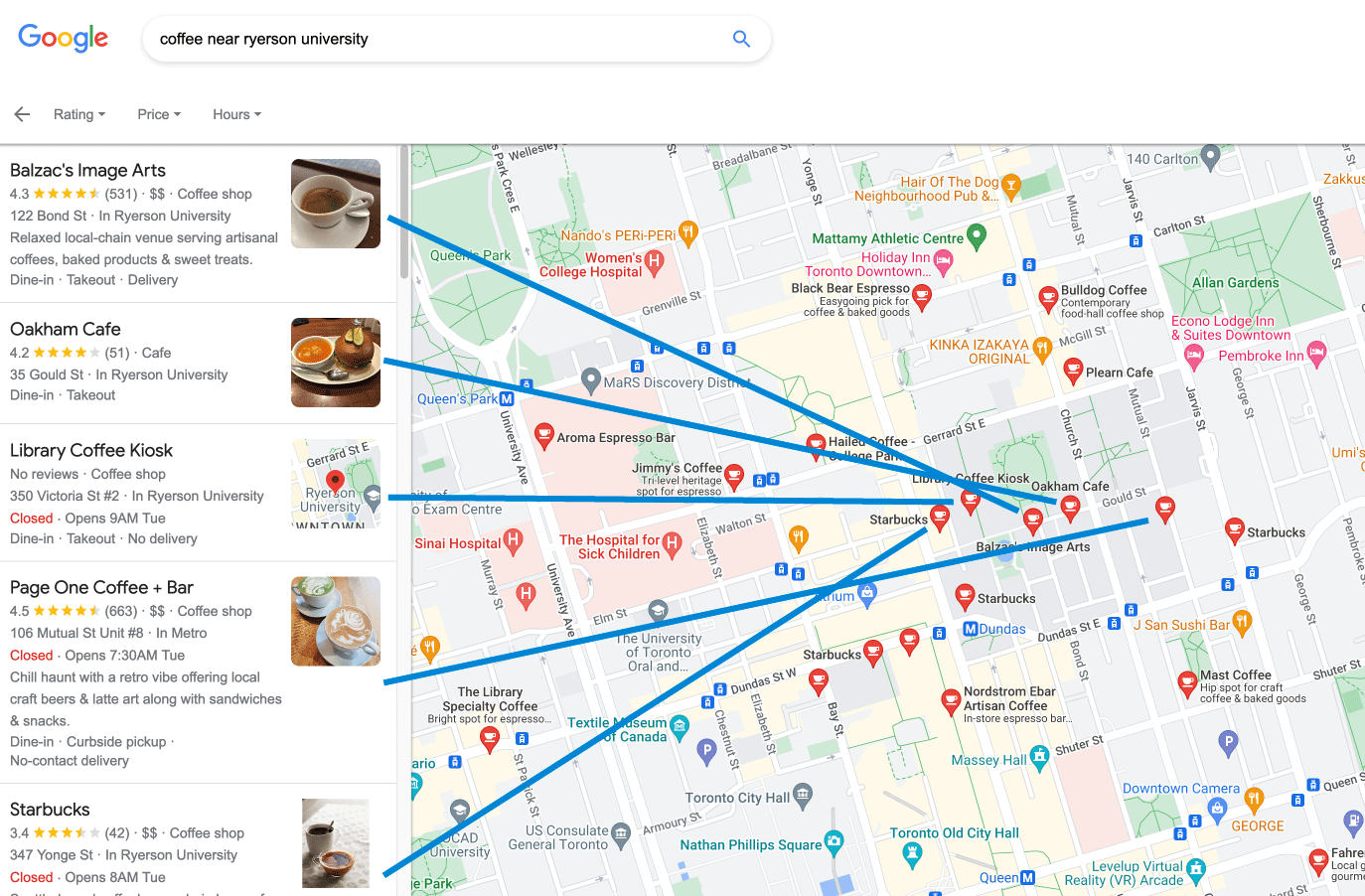This image is a screenshot from Google, showcasing a search for "coffee near Ryerson University." The Google logo appears in the upper left corner, and the search results are prominently displayed on the left side. The top result is Balzac's Image Arts, boasting a rating of 4.3 stars from 531 reviews. It is followed by OCAM Cafe with 4.2 stars from 51 reviews, Library Coffee Kiosk which has no reviews, Page One Coffee Bar with the highest rating at 4.5 stars from 663 reviews, and finally, Starbucks with a rating of 3.4 stars from 42 reviews. Blue lines have been drawn from each coffee shop listing directly to their respective location pins on the map to the right. The map includes pinpoints of the mentioned coffee shops around Ryerson University, as well as other points of interest in the vicinity.